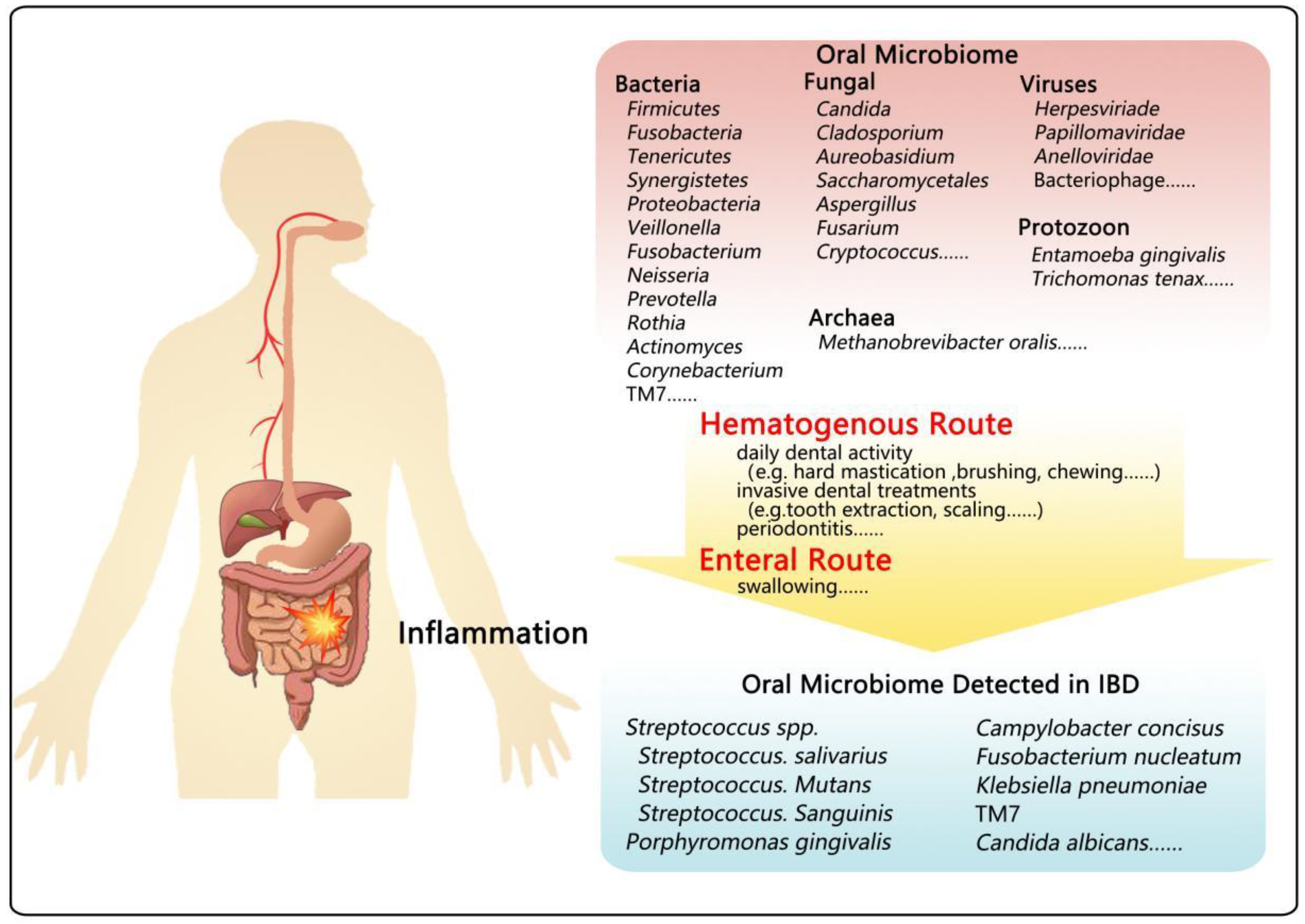This detailed infographic depicts a human silhouette showcasing the internal digestive system. Central to the image is an illustration highlighting the digestive tract, with a dramatic red, orange, and yellow explosive design centered in the intestinal area, symbolizing pain and inflammation. To the right of the silhouette, "Inflammation" is prominently displayed in black font. At the top of the image, the term "Oral Microbiomes" is featured, accompanied by a comprehensive list of various microorganisms including bacteria, fungi, archaea, viruses, and protozoa. Beneath this, the infographic presents "The Hematogenous Route" followed by "The Enteral Route". At the bottom, there is a detailed section titled "Oral Microbiomes Detected in IBD," providing specific listings and classifications under each heading. The visual representation effectively emphasizes the connection between oral microorganisms and intestinal inflammation, particularly in the context of inflammatory bowel disease (IBD).